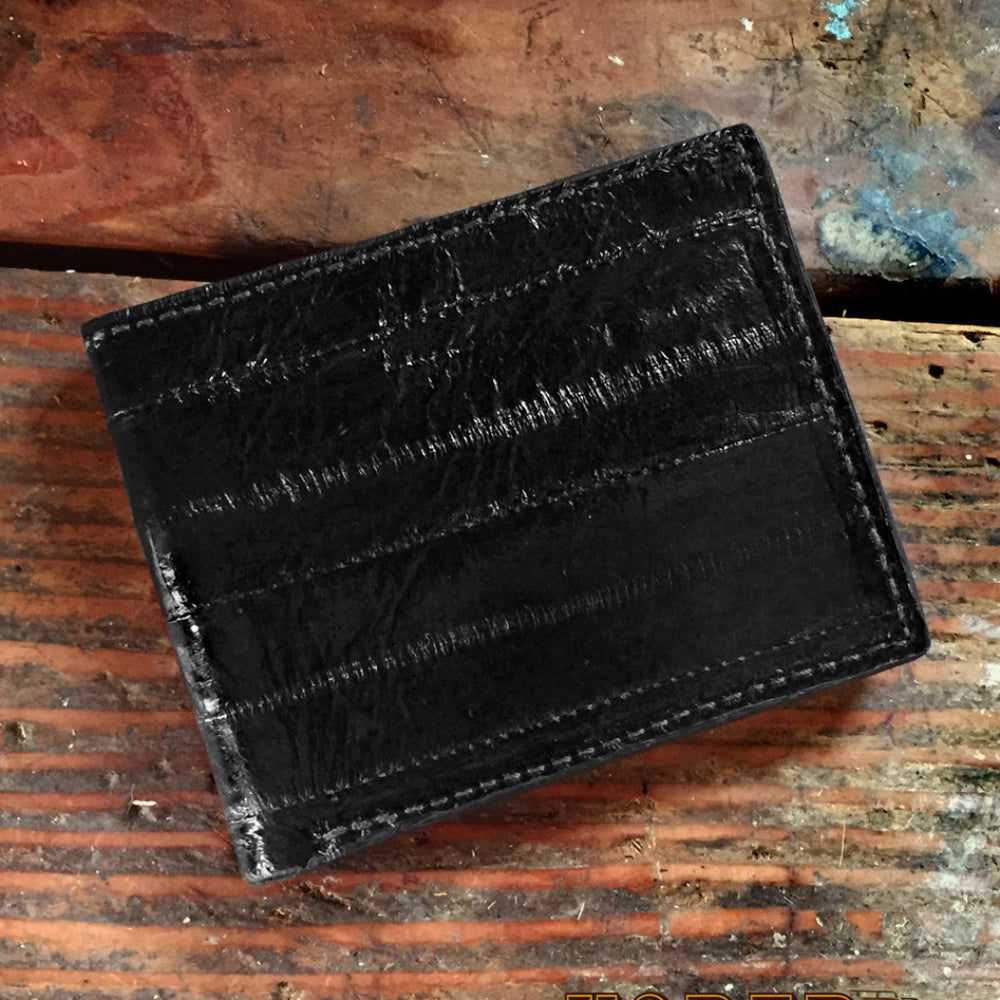The image showcases a promotional product, specifically a black leather wallet with gray stitching, displaying a textured, shiny, and possibly snake or alligator skin-like surface. The wallet, appearing slightly cocked to the left with its opening on the right, is prominently featured on an old, weathered wooden table. The table is heavily stained, featuring a range of dirt and discoloration, including dark stains, raw wood patches, and various white and blue gunk on the top right and bottom right corners. The table’s surface also includes a notable crack near the top and appears to be deteriorating with signs of insect damage and significant dirt accumulation over years.